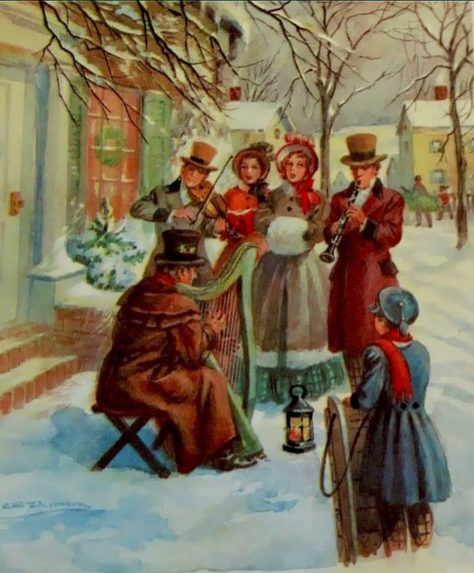This detailed, old-style drawing or painting portrays a festive winter scene reminiscent of the late 1800s or early 1900s, centered around a group of musicians likely performing Christmas carols. The focal point is a seated man dressed in a brown overcoat and black top hat, playing a green harp. Surrounding him are four standing musicians: a man with a violin, another with a clarinet, and two women who appear to be singing. All the figures are attired in period-specific, elaborate clothing; men in top hats and heavy overcoats, and women in voluminous dresses.

A small child, possibly a girl, stands to the right, dressed in a blue coat and hat with a red scarf and a sled nearby, observing the scene. The background features a cozy, snow-covered village with trees devoid of leaves, brick houses, and a prominent home decorated with a Christmas wreath. Snow blankets the ground, shrubs, and rooftops, completing this picturesque Christmas-time vignette.